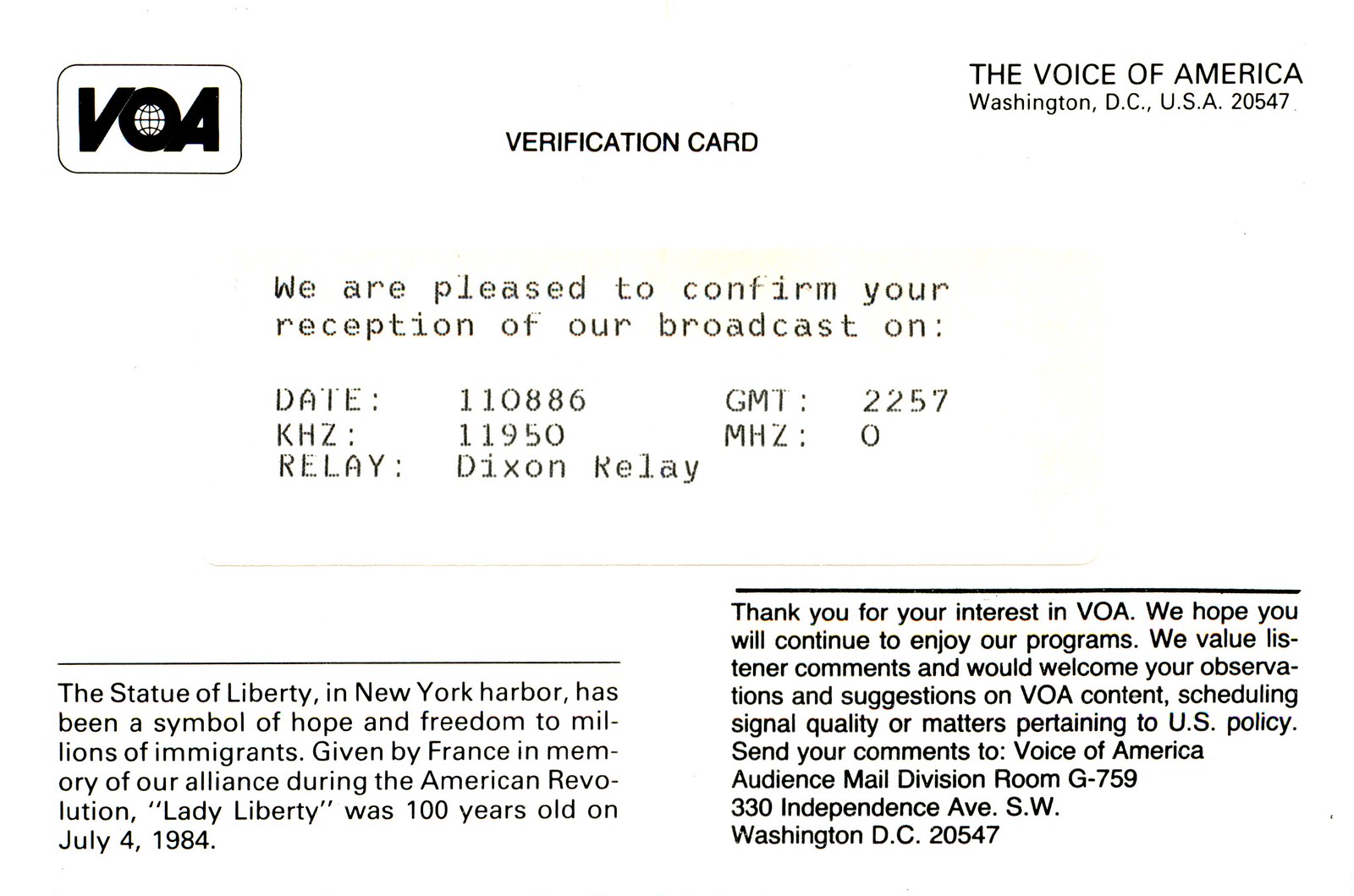This image depicts a vintage QSL verification card from Voice of America (VOA). The card features a black and white logo in the top left corner with the letters "VOA" and a globe symbol embedded within the "O". At the top center, the card reads "Verification Card," and on the right side, "The Voice of America, Washington DC, USA 20547." The main text in the center confirms reception of a broadcast on November 8, 1986, at 22:57 GMT on frequency 11,950 kHz from the Dixon Relay station. Below this, a line of text mentions the significance of the Statue of Liberty, stating: "The Statue of Liberty in New York Harbor has been a symbol of hope and freedom to millions of immigrants. Given by France in memory of our alliance during the American Revolution, Lady Liberty was 100 years old on July 4, 1984." A black line separates this paragraph from the centered text. On the right side of the card, a message thanks the recipient for their interest in VOA, expresses hope that they will continue to enjoy the programs, and encourages listener feedback regarding content, scheduling, signal quality, or related U.S. policy matters. Comments can be sent to the Voice of America Audience Mail Division, Room G-759, 330 Independence Avenue SW, Washington DC 20547. The card has a white background with detailed black text and line art.